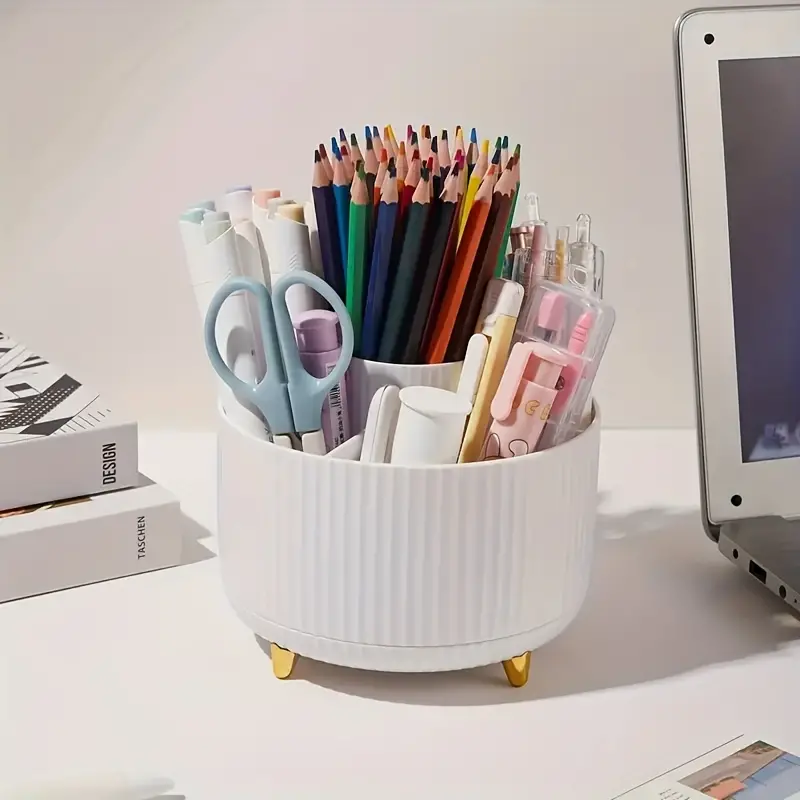The high-quality image is an advertisement for a white ceramic pen organizer with two tiers, elegantly supported by four gold-painted legs. The round, two-tiered ceramic organizer is designed to hold various office supplies, evident by the markers, highlighters, colored pencils, safety scissors with blue handles, and gel pens neatly arranged within its compartments. The central section of the organizer contains colored pencils, while markers and scissors are positioned to the left, and assorted pens fill the right compartment. 

The scene is set on a pristine white desk, with a corner of two design books peeking out on the left side, and an open laptop situated on the right. The backdrop is a smooth, white paper typical of a lightbox setup, creating a seamless and professional appearance. The organizer is prominently displayed, emphasizing its functionality and stylish design, suitable for a well-organized and aesthetically pleasing workspace.